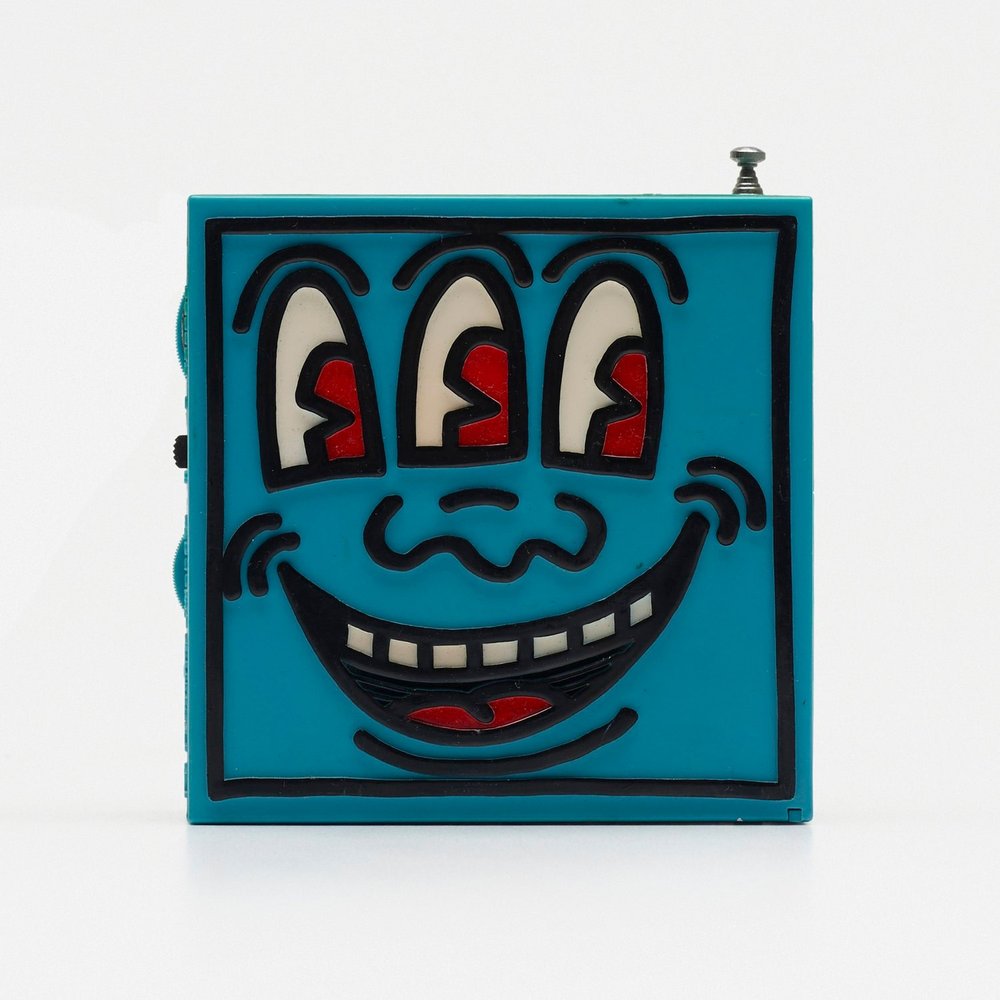The image depicts a turquoise blue plastic box, which resembles a children's toy or a whimsical radio. Prominently featured on the front face, which is bordered by a black square line, is a cartoonish three-eyed smiley face. Each eye has a red iris and is topped by an arched eyebrow. The face includes additional details such as a nose and a wide grin, showcasing seven white teeth and a red tongue, with smile lines at the corners enhancing the jovial expression. At the top right of the box, there is a black 'X' button, possibly a power switch, and on the left side, there is a partially visible blue dial, speculated to be for tuning or volume control. An antenna, retracted fully, extends from the top, hinting at the object's potential as a playful radio.